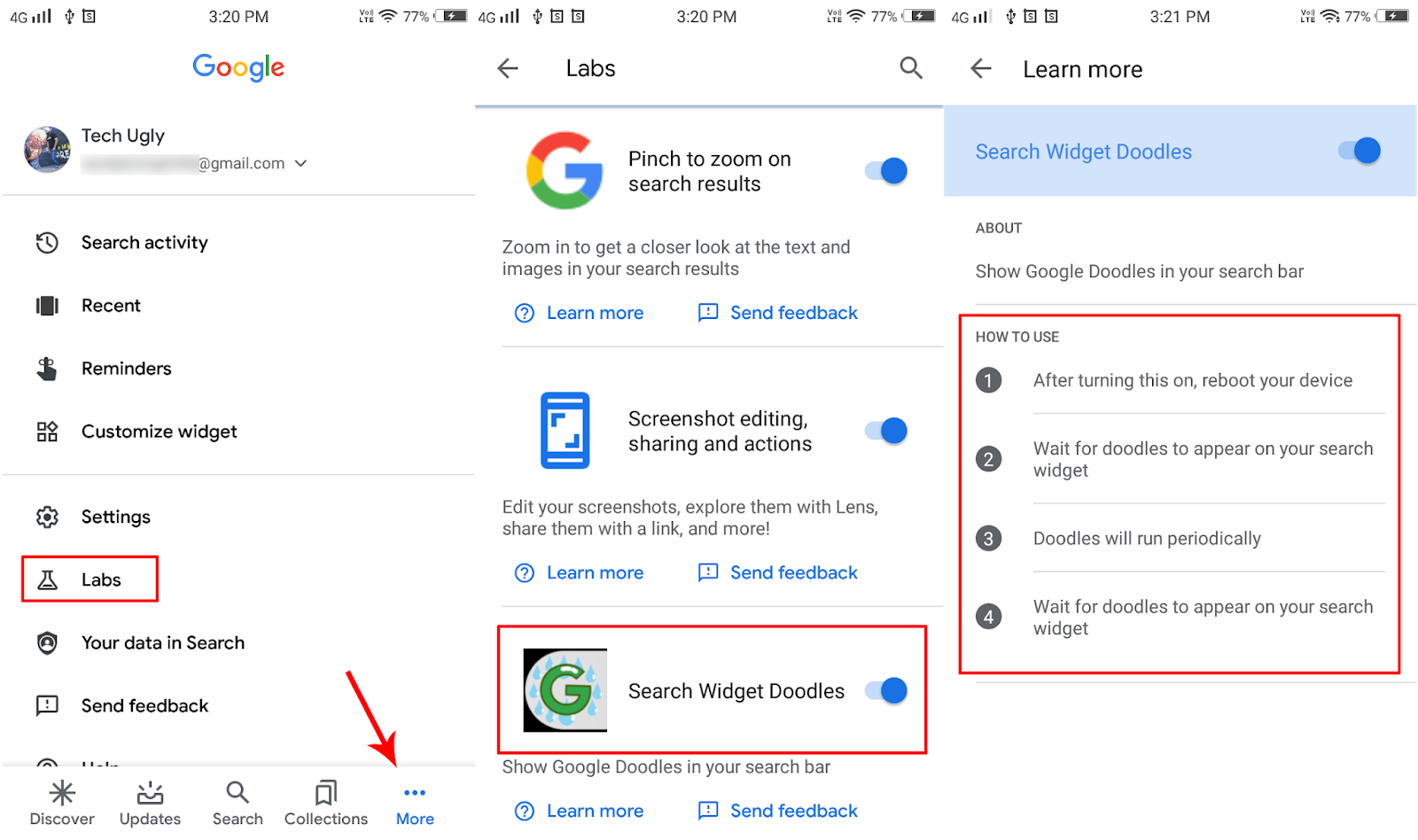The image comprises three different cellphone screenshots. On the left, two screenshots indicate the time as 3:20, and on the right, one shows the time as 3:21. 

**First Screenshot:**
- The email “techugly” followed by a blurred domain is displayed.
- Below the email, options listed are: “Search activity,” “Recent reminders,” “Customized widget.”
- A gear icon labeled “Settings” and a lab beaker icon labeled “Lab” are also visible.
- The section “Your data in search” is highlighted with a red box around it.
- Further options include “Send feedback,” “Discover,” “Update,” and “Search collection.”
- There is a blue hyperlink labeled “More” with an ellipsis and a red arrow pointing at the ellipsis.

**Second Screenshot:**
- The phrase “Pinch to zoom on search results” appears with a toggle bar turned on.
- An additional note says, “Zoom in to get a closer look at the text and images in your search results.”
- Options “Learn more” and “Send feedback” are provided below.

**Third Screenshot:**
- The screenshot mentions “Screenshot editing, sharing, and actions” with an active toggle bar.
- The description reads, “Edit your screenshots, explore them with Lens, share them with a link, and more.”

This detailed caption comprehensively describes the contents and features captured in the screenshots.